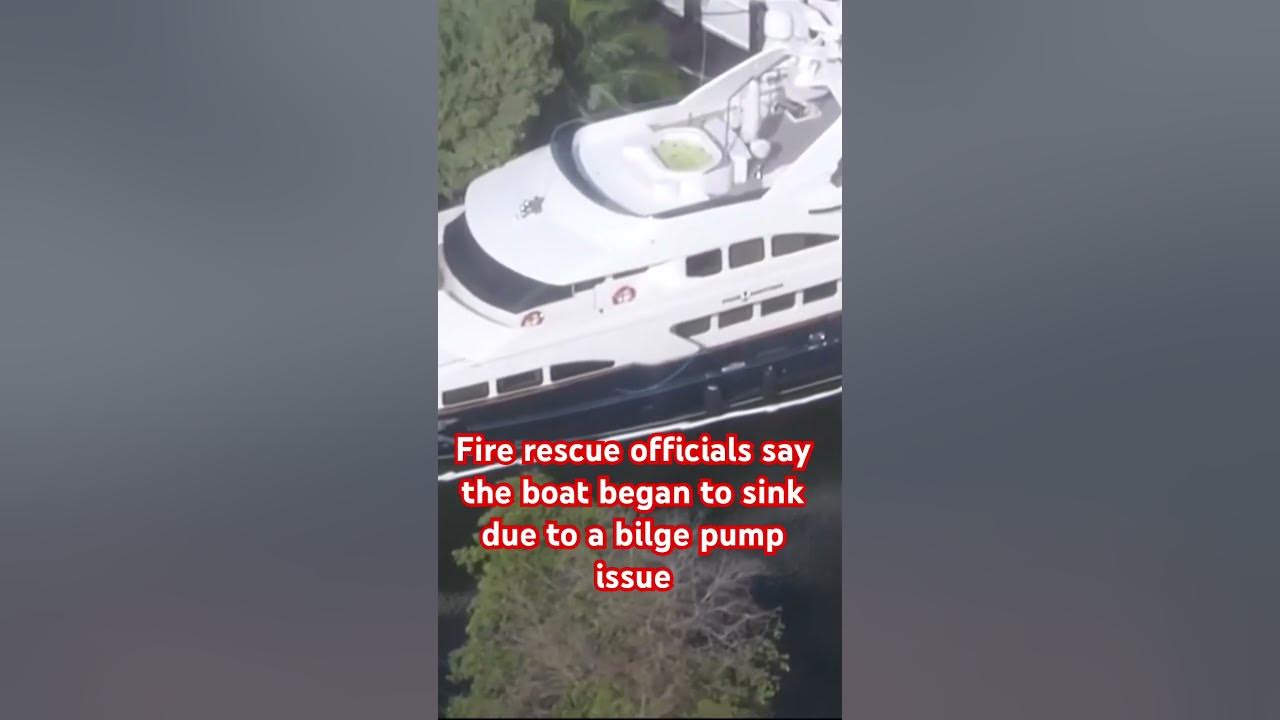This image, clipped from a vertical TikTok or Instagram reel video, depicts a close-up of a large white yacht partially submerged in water. The yacht, situated amidst lush green trees, features a navy-blue hull and several windows—three on the top deck and four on the bottom right side. Text, in white with a red outline, overlays the middle of the image, stating that "fire rescue officials say the boat began to sink due to a bilge pump issue." The photograph captures the midship section, excluding the fo'c'sle, and includes glimpses of a dock and a pool or jacuzzi on the yacht's top deck.